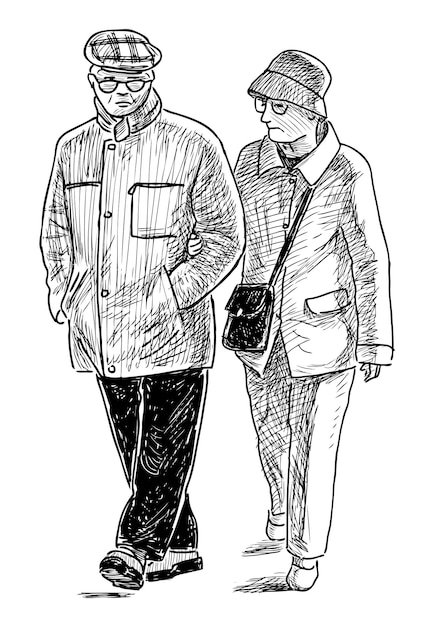This black and white sketch portrays an elderly couple walking together, facing toward the viewer against a plain white background, reminiscent of a winter day. The man, on the left, is depicted with a British-style cap, glasses, a pocketed jacket, and dark pants. His hands are in his coat pockets, and he appears to be taking a step forward. The woman, on the right, also wears a hat and glasses. She has a lighter jacket with pockets at the bottom, and is carrying a dark purse over her shoulder. Her pants appear lighter in color, with shadows sketched in. One of her hands holds the elbow of her partner, showing a gesture of support. Both individuals have somber expressions, with the man looking towards the woman and the woman looking down in his direction.